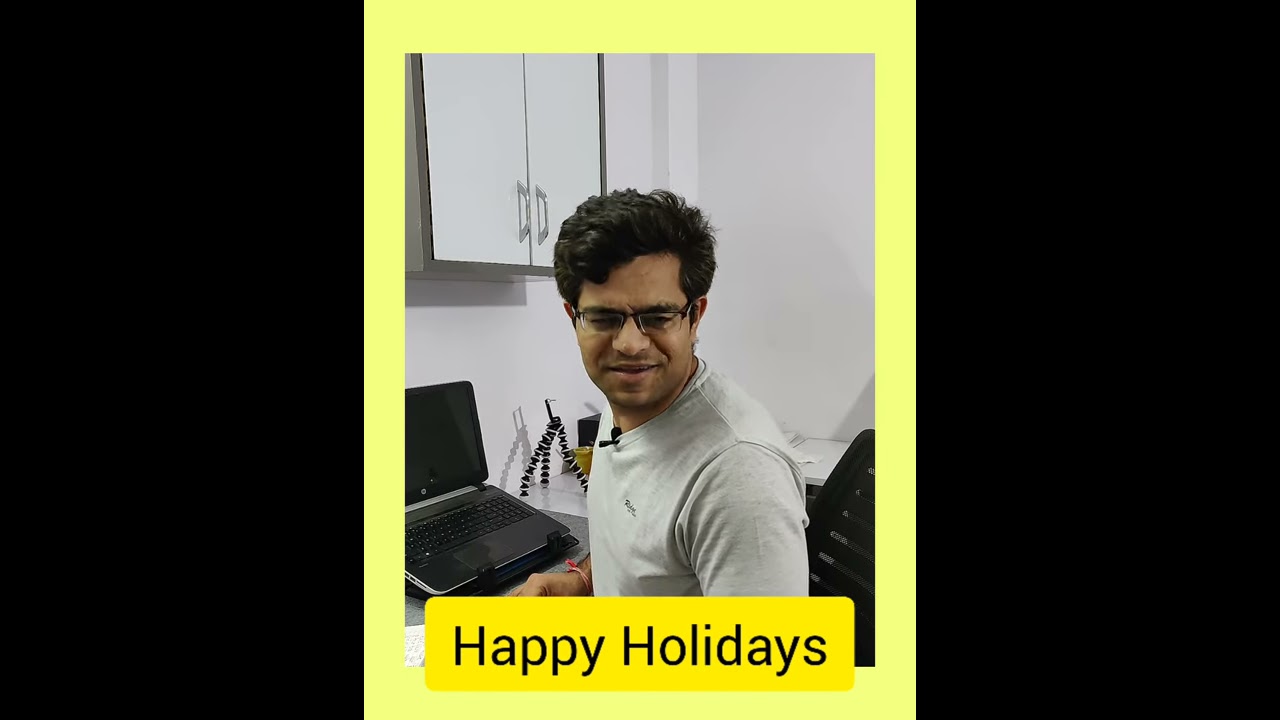A man with short black shaggy hair and black-rimmed glasses is sitting at a white desk in a black leather office chair. He is wearing a light gray, short-sleeved shirt with a logo on the front, and has a microphone clipped to it. He is smiling with his eyes slightly closed and looking away from the angled black laptop sitting on a silver mat on the desk. His right hand, adorned with a bracelet, rests on the desk next to the laptop, which is propped up by a stand. On the desk are several objects, including a tripod and what appears to be a piece of artwork with three prongs, along with a tissue. Behind him is a white wall with attached white cabinetry with gray handles. The image is framed by a thick yellow border, and a yellow rectangular text box at the top of the image has "Happy Holidays" written in black. This framing and text suggest that the image serves as a holiday card. The entire picture is centered on a rectangle with blacked-out left and right sides.